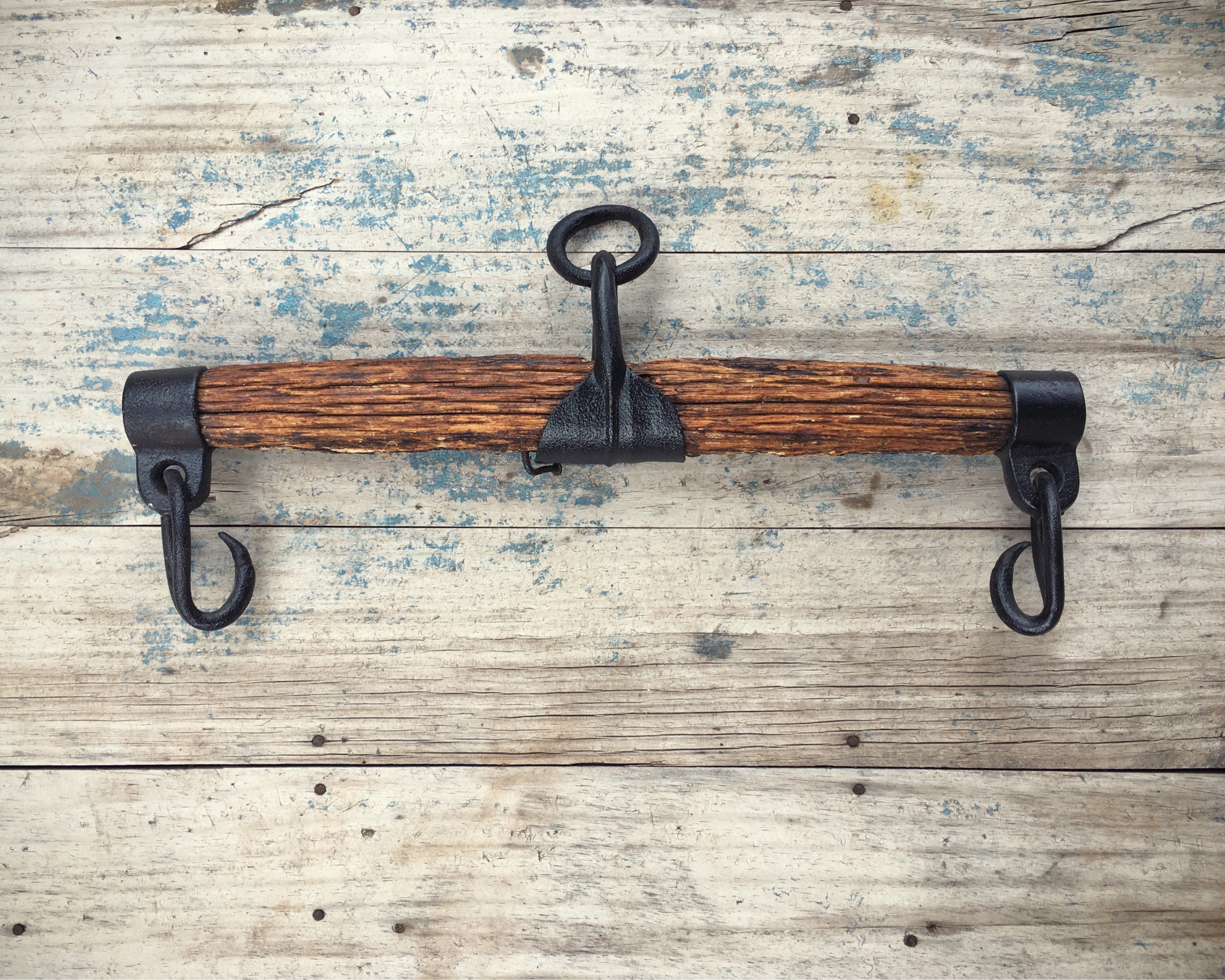The full-color, square photograph has a clearly staged setup, where the background is composed of weathered wooden boards with remnants of old blue paint mostly washed off. The wood appears very dry and cracked, and nail holes as well as actual nails are visible, particularly towards the bottom. The overall tone of the wood gives an aged look to the setting.

In the center of the image runs a horizontally positioned piece of antique farm equipment. This piece of wood, appearing very aged and worn, spans about two to three feet. Both ends of this wooden beam are capped with what look like large, black, cast-iron fittings. Each of these fittings has a significant hook extending from it, with the right hook curving to the left and the left hook curving to the right.

Wrapped around the center of the wooden beam is a black metal ring, from which a post extends upward, culminating in an O-ring on top—perhaps designed to allow the apparatus to hang from a wall. The entire setup suggests it might be an old yoke or harness, potentially used for attaching animals like horses or cows to a carriage or for farm work pulling equipment.

It's not entirely clear if the photograph was taken indoors or outdoors due to the uniform, nondescript wooden background. However, the detailed description of the worn and cracked wood, hints at its long exposure to the elements, enhancing its historical and rustic aesthetic.